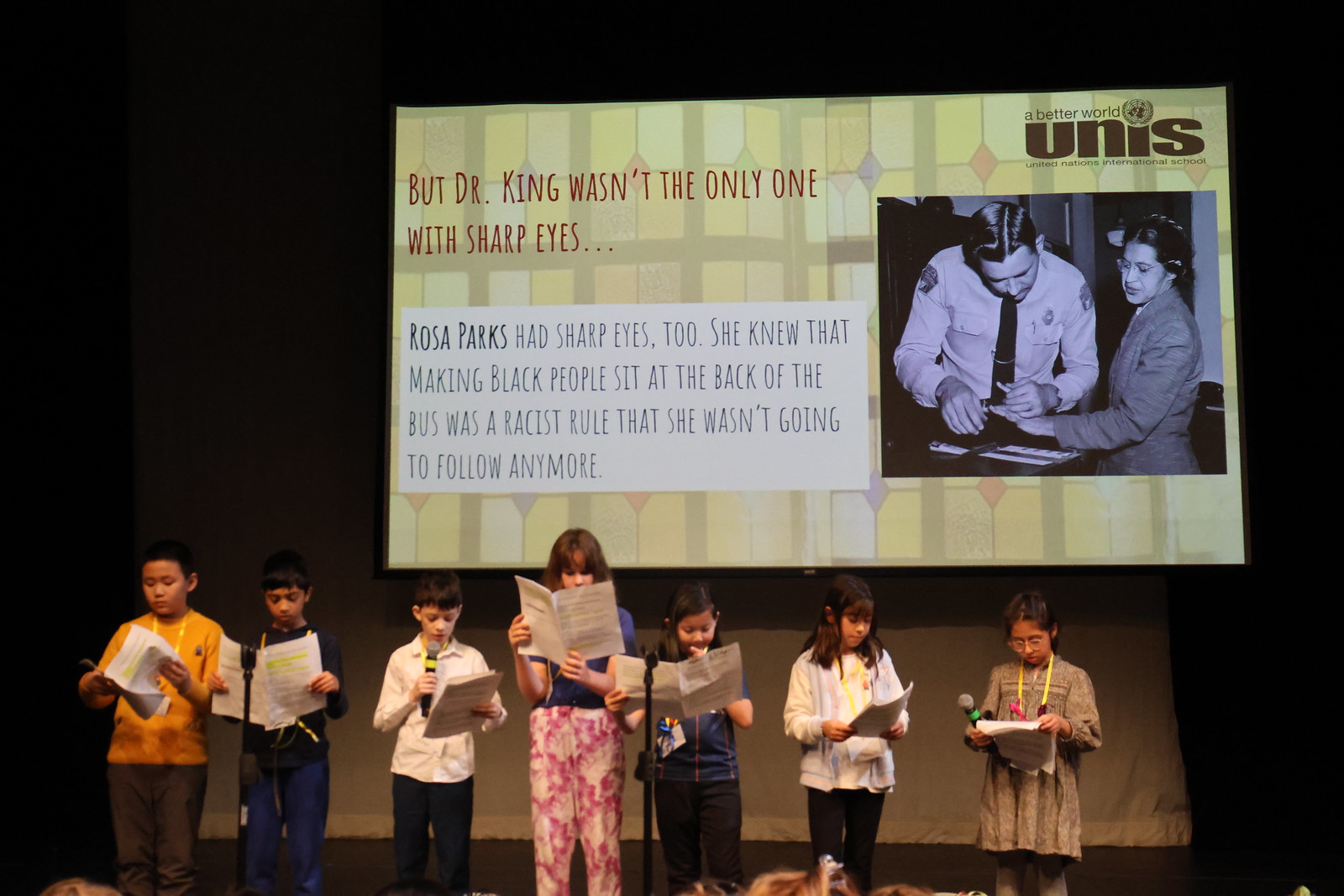In this color photograph, a group of seven children, both boys and girls, are standing on a stage, appearing to participate in a performance or reading. Each child holds a white pamphlet, some with highlighted yellow sections, and they are taking turns reading aloud to an audience. Notably, the third child from the left is holding a microphone. The children are dressed in various colorful outfits, including an orange shirt and pink pants among others, adding a vibrant touch to the scene.

Behind the children, a large screen displays a slide used for their presentation. The slide features a prominent black and white photograph likely depicting Rosa Parks being fingerprinted, linking it to her historic act of defiance against racial segregation. To the upper right of the screen, there is a logo that reads "A Better World, UNES." To the left, red text states, "But Dr. King wasn't the only one with sharp eyes," followed by a smaller patch of white with black text underneath, stating, "Rosa Parks had sharp eyes too. She knew that making black people sit at the back of the bus was a racist rule that she wasn't going to follow anymore." The setting appears to be inside a hall, classroom, or auditorium, emphasizing the educational and historical nature of the event.